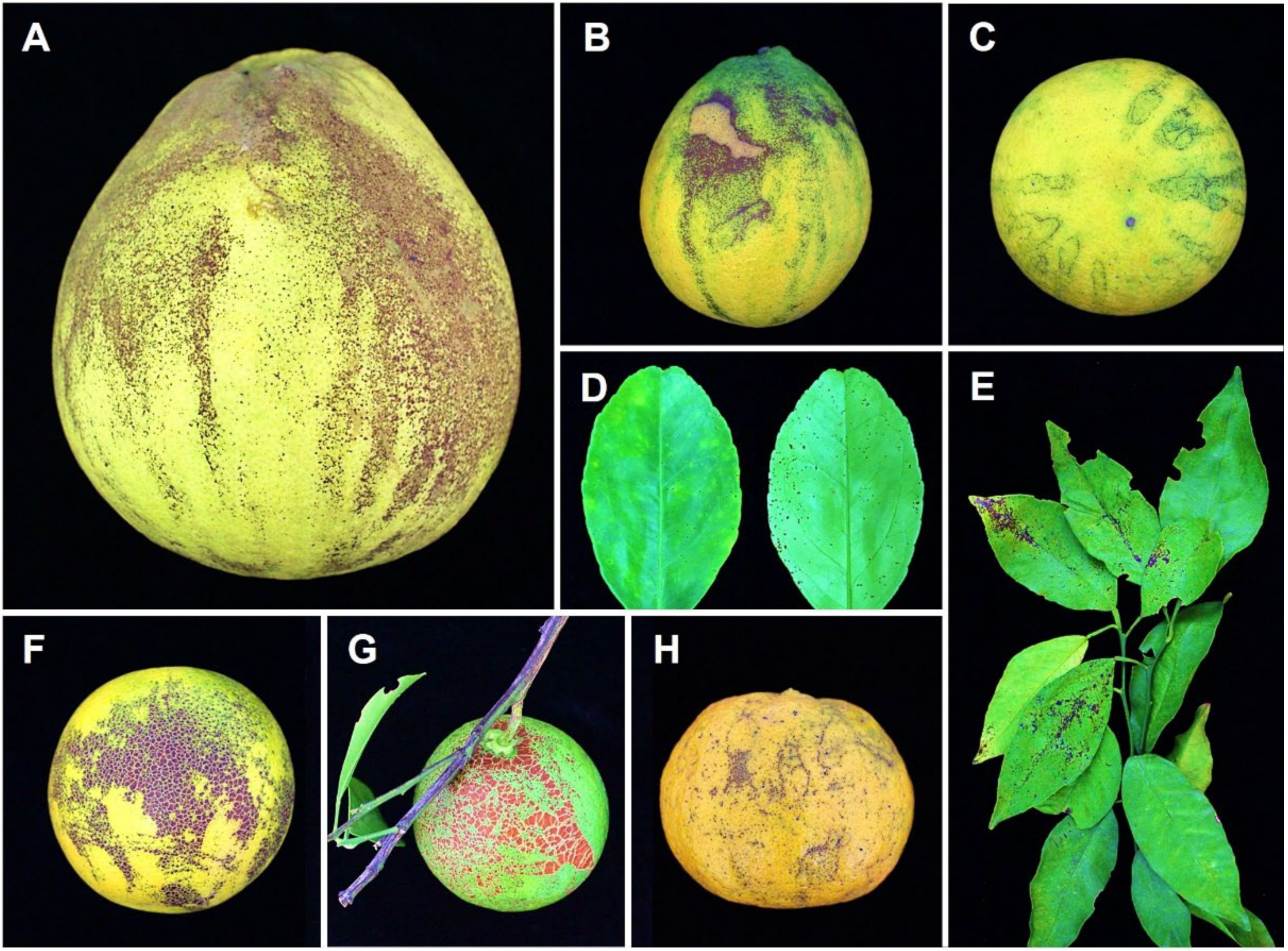The image showcases a grid of various fruits and leaves arranged within black panels, each labeled with letters from A to H along the top left corner. Each panel contains a distinct fruit or leaf with unique characteristics described as follows:
- **Panel A**: Features a yellow fruit with a brownish finish.
- **Panel B**: Shows a green fruit with a small brown spot.
- **Panel C**: Displays a round, greenish-yellow fruit.
- **Panel D**: Contains two green leaves.
- **Panel E**: Highlights a cluster of green leaves.
- **Panel F**: Contains a ball-shaped, yellow fruit marked with dark spots.
- **Panel G**: Holds a green fruit adorned with red spots and includes a small branch with a leaf.
- **Panel H**: Features an orange fruit dotted with black spots.

Each fruit and leaf is distinct in color, shape, and texture, providing a detailed visual exploration of botanical diversity within the grid.